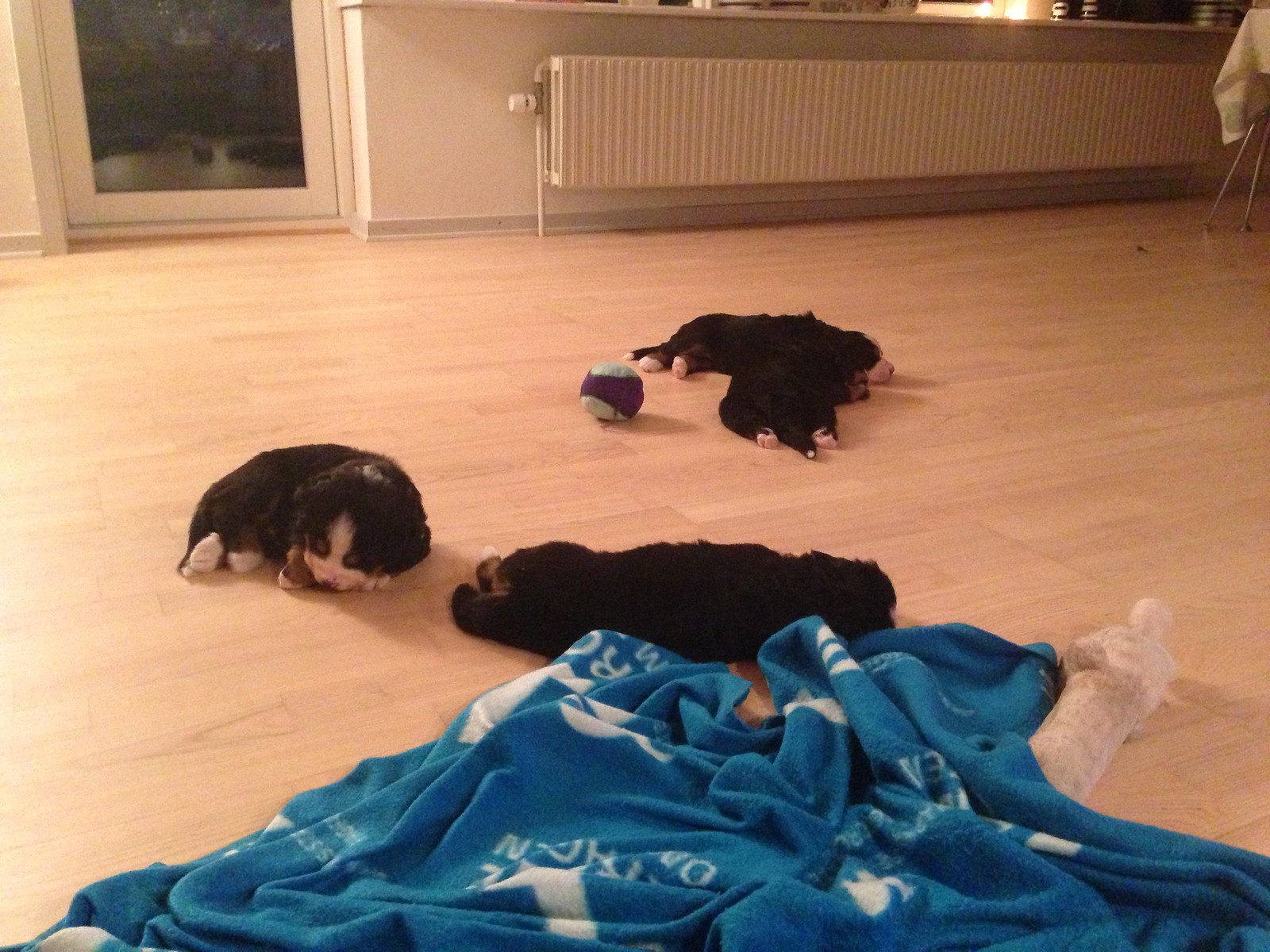This image captures a cozy indoor scene featuring four adorable puppies sound asleep on a light-colored, blonde hardwood floor. Their bodies are mostly dark with some distinctive white markings on their paws, faces, and tails. The puppies are comfortably spread out, with two lying close together and the other two positioned individually closer to the photographer. 

In the foreground, a crumpled blue and white patterned blanket adds a touch of softness, and a white stuffed toy peeks out from underneath it. A teal and white stuffed ball lies by one of the puppies in the center of the arrangement. Behind the group, a long, raised radiator runs along the tan-colored wall, while an open room stretches out with a table draped in a tablecloth positioned towards the back. The room also features a full glass door on the left, hinting at the dark outside. Just above the radiator, a counter or ledge extends with two lights, subtly illuminating the peaceful scene of puppies, content and resting after what seems like a playful day.